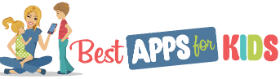In the image, a vibrant, cartoonish scene captures a warm, family-friendly moment. At the center, a blonde woman with short hair—or perhaps it is pulled back—sits comfortably on the floor. She is dressed casually in a blue shirt, blue jeans, and navy shoes. On her lap, she holds a young girl with matching blonde hair tied back in a ponytail. The girl is adorned in a charming green and white polka-dotted outfit, gazing with interest at the smartphone her mother is holding.

Standing beside them is a young boy with brownish hair, donned in a bright red shirt and teal pants, looking curiously at the screen. The mother’s focused yet gentle expression suggests she is deeply engaged in showing the children something on her phone, creating a scene filled with warmth and connection.

Above this delightful tableau, the words “Best Apps for Kids” are prominently featured. "Best" is written in a playful red cursive font. Below it, a white rectangle boldly displays “APPS” in all capital letters. The word “for” is rendered in cursive green, bringing a touch of elegance to the design. Finally, “KIDS” stands out in all capital letters, with each character a different vibrant color: the K in red, I in teal, D in green, and S in red.

The composition seamlessly blends the familial and educational atmosphere, emphasizing the theme of the best apps designed for children.